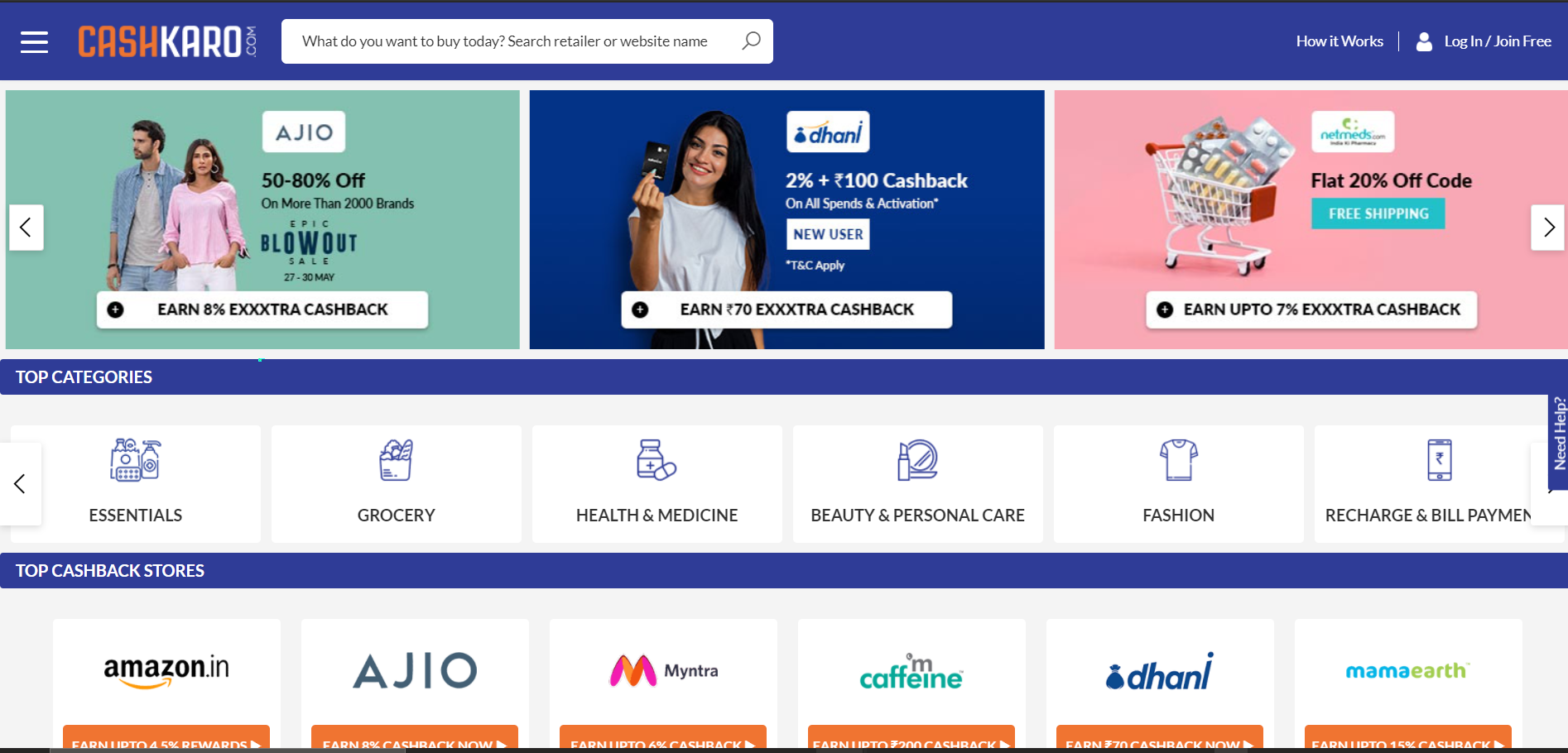**Screenshot Description:**

The screenshot captures the homepage of the website "cashcard.com." 

**Header Section:**
At the very top, the header includes three menu options. To the right of the menus, the website name “cashcard.com” is prominently displayed. Next to this, there is a search bar followed by a section on “how it works” accompanied by an icon of a person. Towards the far right of the header, there is an option to "Login" or "Join Free."

**Main Content:**
Directly below the header are three promotional rectangles offering various deals and cashback options:

1. **Left Rectangle (Green Background):**
   - **Visual:** A picture of a man and a woman.
   - **Text:** "Agio 50-80% off – Blowout. Earn extra cashback."

2. **Middle Rectangle (Dark Blue Background):**
   - **Text:** "D hard. Get 2% + ₹100 cashback if you're a new user. Earn ₹170 extra cashback."

3. **Right Rectangle (Pink Background):**
   - **Visual:** A shopping cart.
   - **Text:** "Flat 20% off code and free shipping. Earn up to 7% extra cashback."

**Category Buttons:**
Below the promotional offers, there are buttons for different top categories. These include:
- Essentials
- Grocery
- Health and Medicine
- Reality and Beauty (likely a typo, should be "Beauty")
- Personal Care
- Fashion
- Recharge and Bill Payments

**Top Cashback Stores:**
Further down, there is a list of top cashback stores which includes:
- Amazon India
- Agio
- Myntra
- Caffeine
- Donnie
- Mama Earth